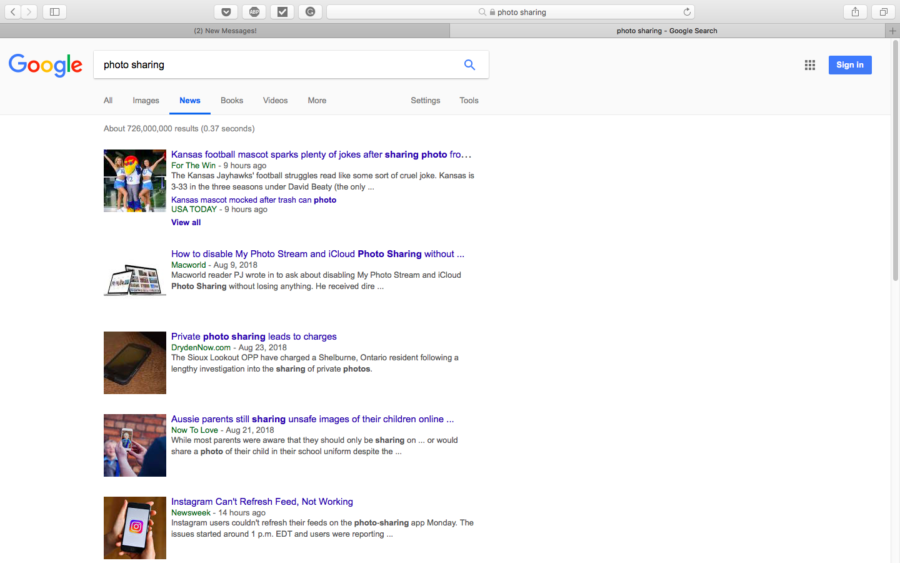This is a comprehensive screenshot of an internet browser, likely Safari. At the top, the grey navigation bar features several control icons on the left: a back arrow, a forward arrow, and a minimize button. Adjacent to these, there are four small grey boxes with unknown icons. The central search field contains the text "II photo sharing". At the end of the search field, a refresh arrow is visible, and in the top-right corner, two more buttons are present—one for minimizing and another for sharing.

Below the navigation bar, there are two open tabs. The tab on the left reads "Two new messages!" while the active tab on the right is titled "photo sharing - Google Search". The main content of the screenshot displays a Google search results page. The background is primarily white with an off-white bar at the top. This bar contains the Google icon on the left followed by another search field pre-filled with "photo sharing", marked by a magnifying glass icon at its end.

To the right of the search field, a prominent blue "Sign in" button with white text stands out. Below this section, the interface features navigational options: All, Images, News, Books, Videos, and More, with the "News" category currently selected.